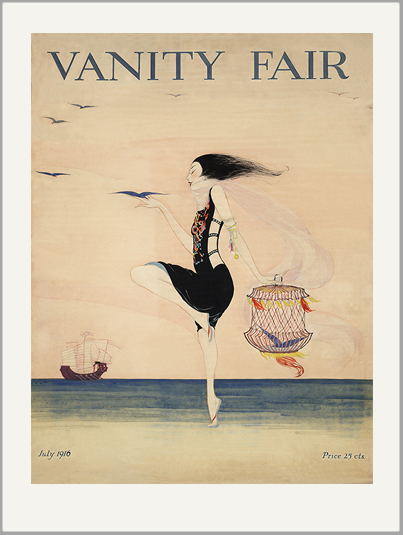This detailed cover of Vanity Fair magazine from July 1916, priced at 25 cents, features a striking drawn image of an Asian woman on a beige-tan, possibly wrinkled background. The woman is elegantly poised on one leg in a ballerina-like stance, wearing a black swimsuit adorned with colorful patterns. Her sleek black hair and very small eyes and eyebrows add to her distinct appearance. She holds a cage with a blue bird in one hand, raised gracefully in the air, while several other birds, varying in grayish-blue hues, seem to flutter around her. In her other hand, she carries a vivid, oriental lantern colored in red, yellow, and blue. The setting is a beach with brownish sand that seamlessly blends into a similarly colored sky. In the far distance, the deep blue sea contrasts sharply, highlighted by a small brown boat with white sails, creating an impression of depth in the serene coastal scene.